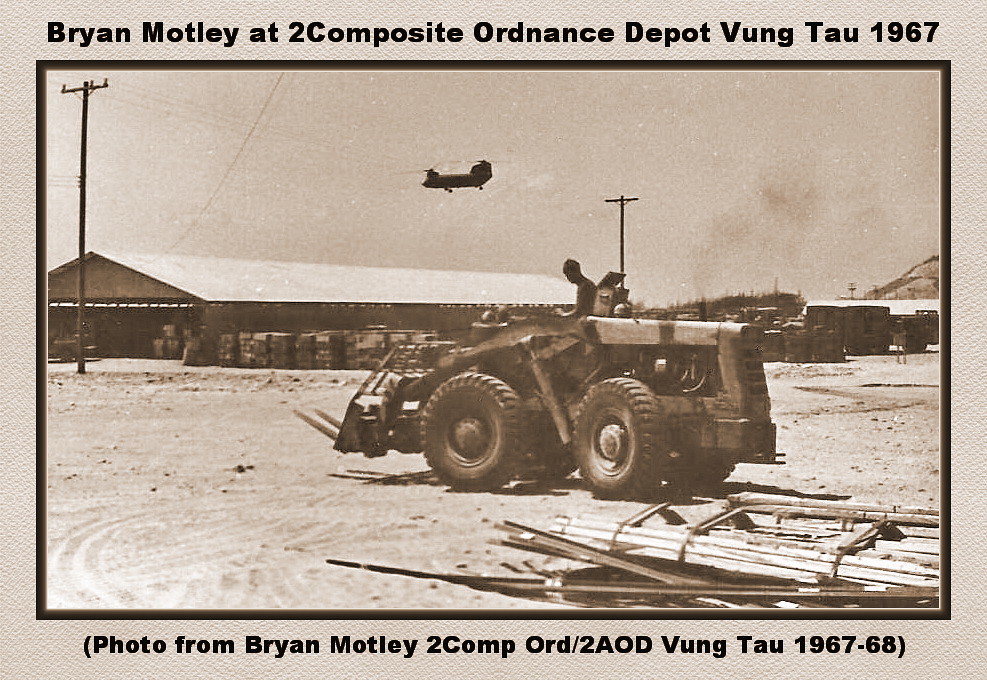The image is a vintage sepia-toned photograph from 1967-68, mounted with a black border and a cream background. The scene, likely at a military base in Vung Tau, shows a man operating a large tractor-like vehicle in a sandy, open field. To the left, a massive hangar is visible with various crates and packages scattered around. Overhead, a plane or helicopter appears as a dark silhouette in the sky. Utility poles with telewires can be seen in the foreground. The photograph features black text at the top and bottom; the top reads: "Brian Motley at 2 Composite Ordnance Depot, Vung Tau, 1967," and the bottom in parentheses states: "Photo from Brian Motley, 2 Comp Ord / 2 AOD, Vung Tau, 1967-68."